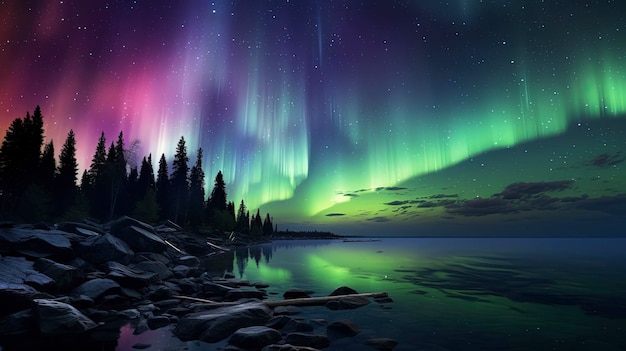This horizontal digital artwork rendering of the Aurora Borealis captures a breathtaking celestial event, showcasing photorealistic detail. The sky is illuminated with dynamic colors transitioning from magenta and pink on the left to purples and blues in the center, and finally vibrant greens fading to yellow on the right. These vivid hues of the Northern Lights are reflected on the serene surface of a lake, enhancing the ethereal quality of the scene. On the left side of the image, a rugged rocky coast is visible, accompanied by a thick line of dark silhouetted pine trees that gradually descend in height towards the right. In the near foreground, a large fallen tree or branch juts out into the water, adding a touch of natural realism. Above the horizon, the effervescent lights of the Aurora blend with scattered stars and a few clouds, creating a mesmerizing and otherworldly night sky.